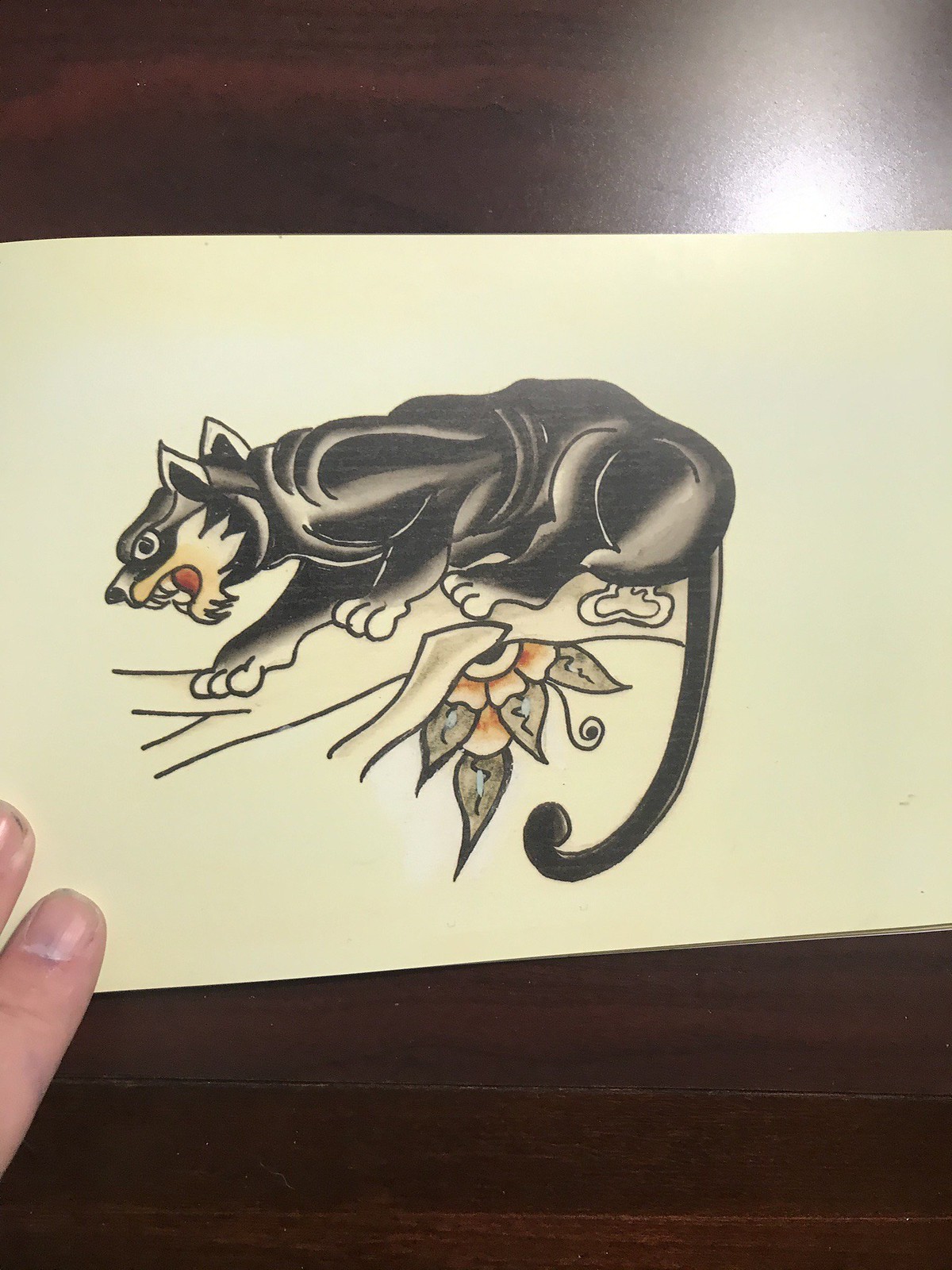In this detailed drawing, a black cat creature is meticulously illustrated on a white piece of paper, which rests atop a dark wooden table illuminated by overhead light. The cat has a strikingly long tail with a distinctive curved end and a face surrounded by golden fur. Its snarling expression reveals a hint of menace, accentuated by a small beard hanging from its chin and wide-open eyes. The cat's feet are depicted in white, contrasting with its dark body. Below the creature, there is a delicate pink flower with gray leaves, providing a splash of color to the composition. Interestingly, there are lines across the drawing, suggesting that the cat might have scratched the surface it is depicted on. A person’s forefinger and middle finger gently touch the drawing, adding a sense of interaction and scale to the scene.